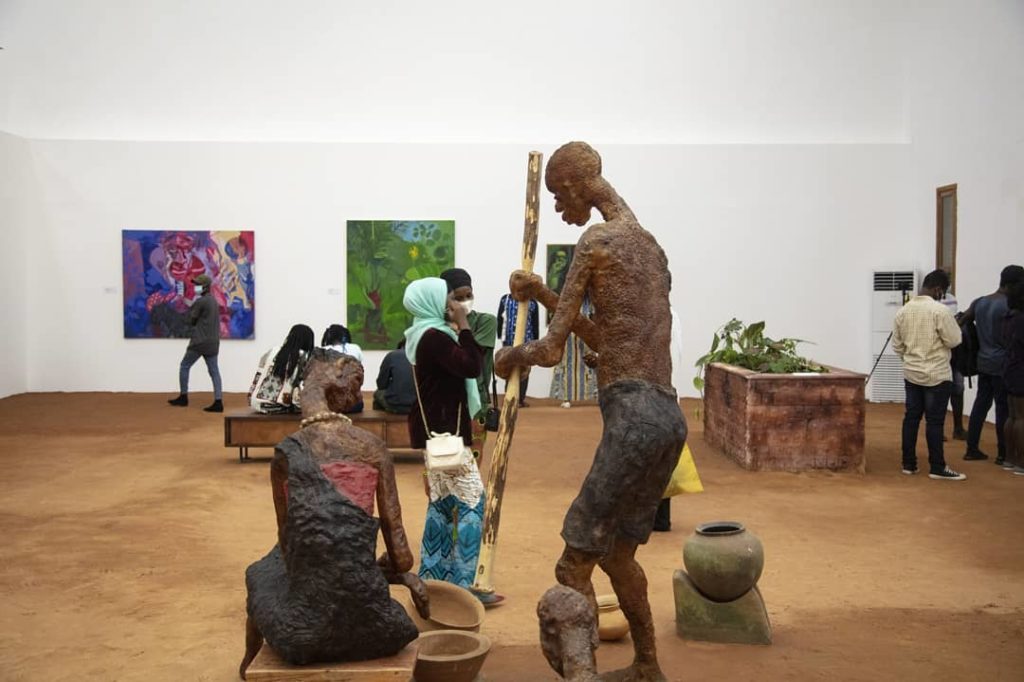This detailed photograph showcases the interior of an art museum or gallery. The floor of the exhibit is covered in brown dirt, mimicking a natural environment. Central to the exhibit are intricate statues that appear to be made of stone or clay. These statues depict African figures, with a male figure holding a long stick or pole, and a female figure seated on a bench, holding a clay pot. Both figures are dressed in traditional African attire, with the male in black shorts and the female in a black dress adorned with a necklace. Behind these statues, the museum's white walls are adorned with three abstract paintings. Visitors, dressed in black, green, and white, are seen walking around and engaging in conversation. Some are observed in the far background, likely admiring the paintings, while others are near the central display, examining the statues and carvings. Additionally, there is a box with plants growing out of it situated in the middle of the room, adding to the exhibit's earthy aesthetic. The overall scene captures the blend of cultural sculpture and contemporary art, with visitors deeply immersed in the experience.